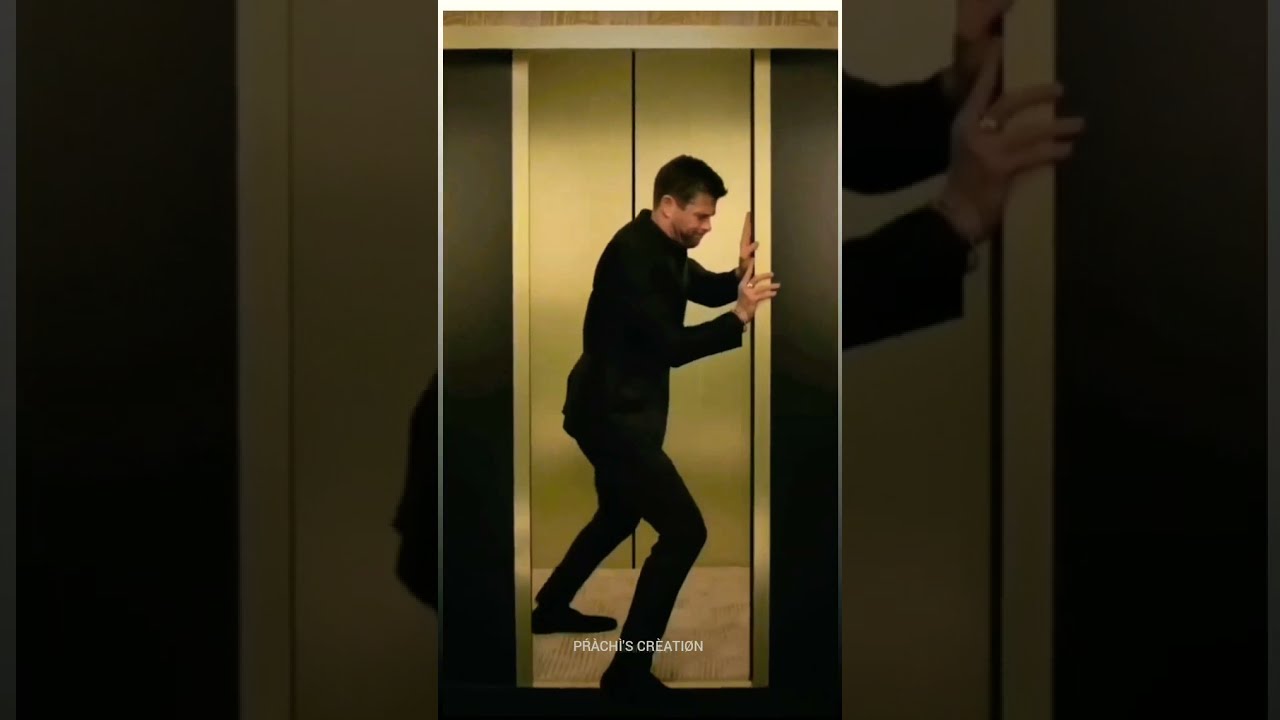The image depicts a light-skinned man with short dark hair, dressed in an all-black outfit consisting of a long-sleeved shirt, pants, and black shoes, inside an elevator. Positioned mostly within the elevator, he uses both hands and his body to brace and push against the right door, with his right foot outside and his knees bent for leverage, trying to prevent it from closing. The elevator features a brown door with gold accents and a matching gold interior with a brown floor. At the bottom of the image, in white text, it reads "Prachi's creation." The original portrait image is extended into a landscape format, with semi-transparent black layers on both sides showing enlarged, detailed segments of the man's hands on the left and part of his back on the right.